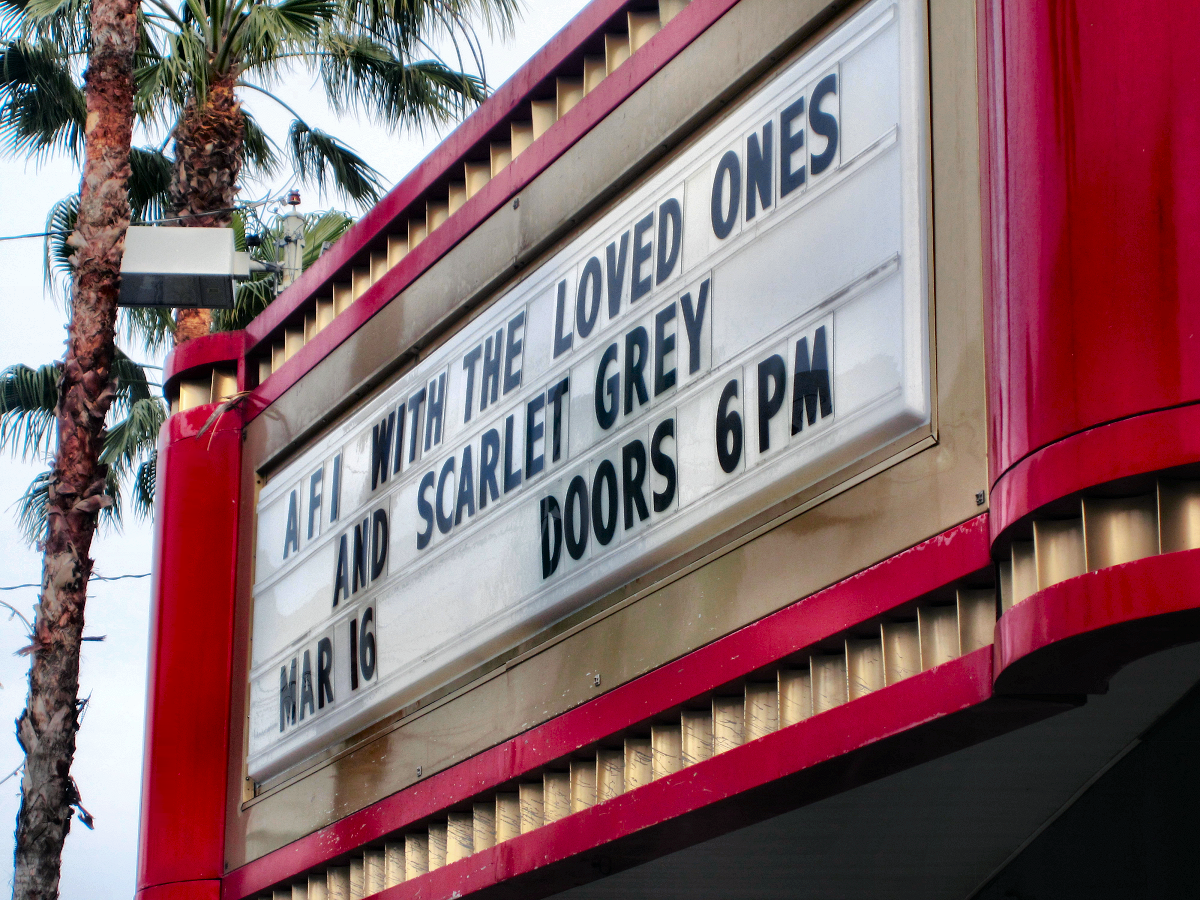The photograph captures the exterior of a building prominently featuring a classic theater marquee overhang. The marquee, which is predominantly red and gold with a corrugated gold border on both the top and bottom, displays the text: "AFI with The Loved Ones and Scarlet Grey, March 16, doors 6 p.m." in black letters on a white display board. The building itself has a striking red and green facade and is accented with a grey light fixture near the left side, next to two tall palm trees. In the background, the bright white sky contrasts with the slightly black lower portion of the building, adding depth to the overall scene.